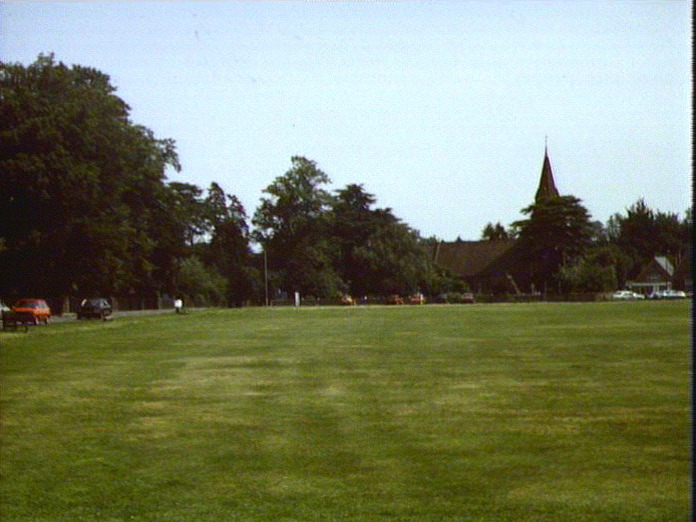This image captures a large, flat grassy field predominantly taking up the bottom half of the frame. The grass is mostly green with occasional patches of white and brown, suggesting a well-trodden or slightly worn area that might resemble a soccer field. A road runs along the left side of the field, lined with both moving and parked vehicles, notably a red car and a black car. The boundary of the field transitions into a backdrop of trees, which are vividly green, adding a natural enclosure to the scene. In the background, beyond the road, a building that appears to serve as a meeting area, possibly even a church given the presence of a steeple-like structure, is visible. The sky overhead is clear and light blue, spanning the upper portion of the image and contrasting gently with the green expanse below. The setting is tranquil, with colors spanning green, brown, tan, red, and blue, thus creating a serene depiction of a suburban or rural landscape, primarily focused on the open grassy area and the peripheral elements that frame it.